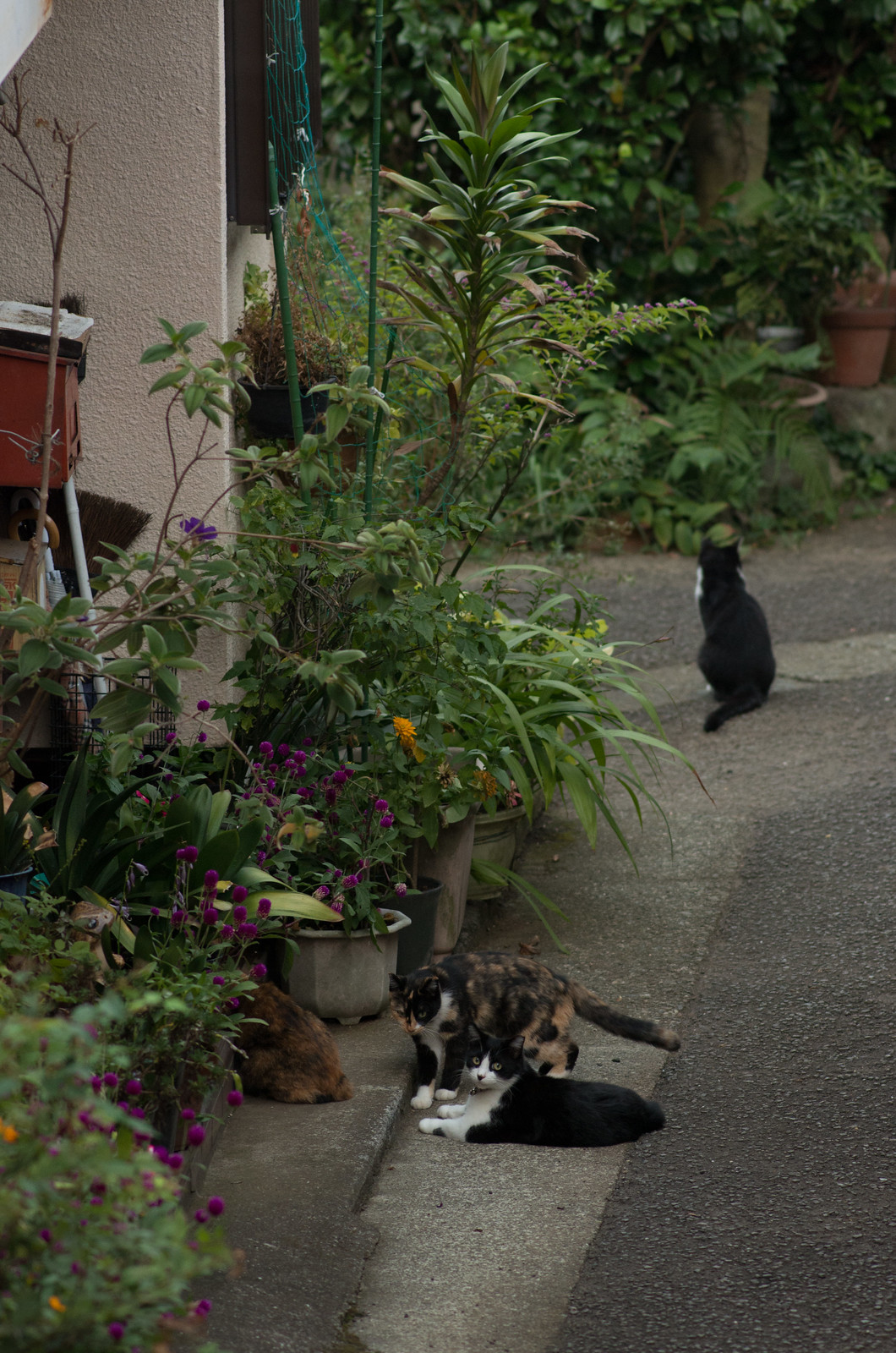This is an outdoor photo taken near the side of a house, showcasing a garden with a variety of plants in pots, some reaching up to four or five feet high. The garden features homegrown plants, including large vines and small ones with purple flowers, creating a nursery-like atmosphere with lush greenery and an abundance of foliage. In the garden, you can see four cats positioned in the scene. At the front, there are three cats: one black and white, one calico, and one brown. The black and white cat is staring directly at the camera, while the calico and brown cats are nearby. In the background, a fourth cat with a black body and a hint of a white neck is facing away from the camera. The garden is bordered by a concrete path and wall, adding a structured element to the vibrant and natural setting.